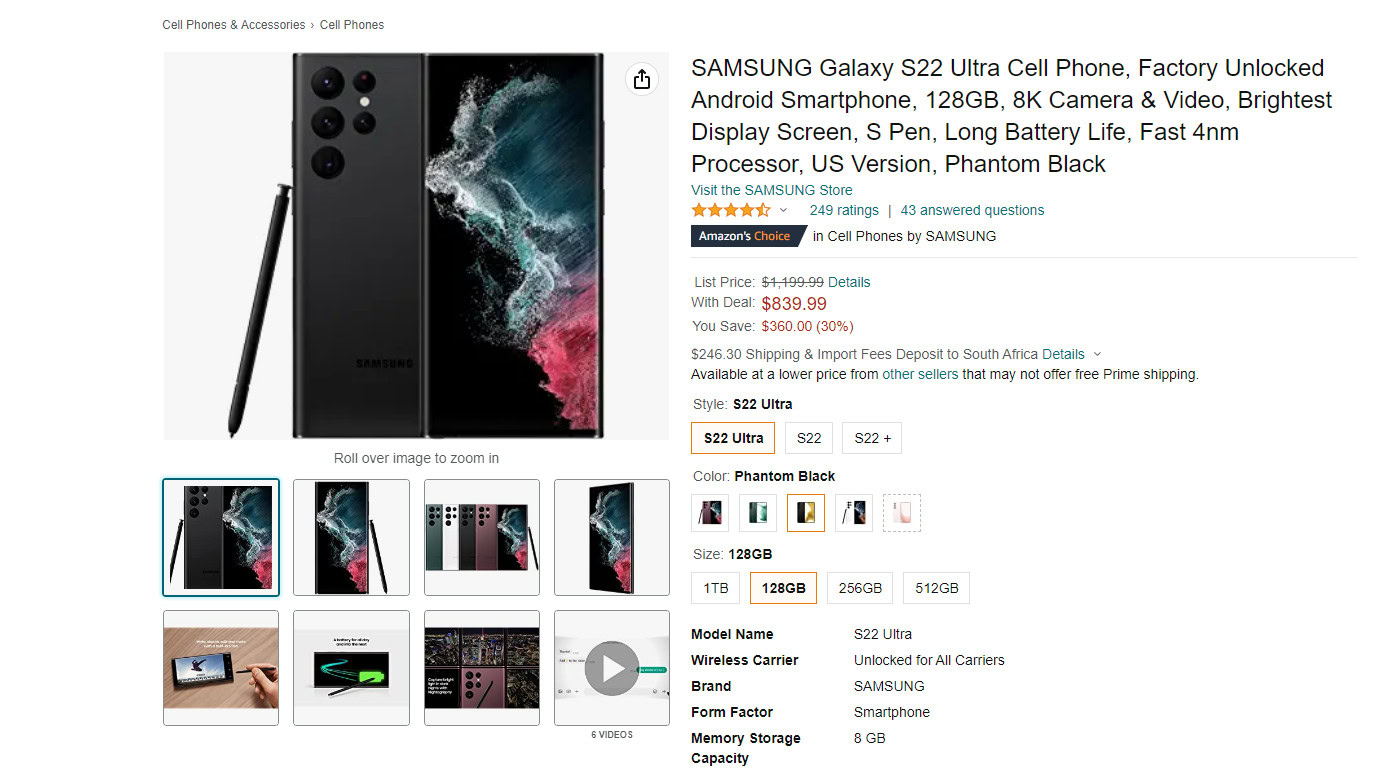**Caption:**

The image is a screenshot from an Amazon product listing, characterized by a predominantly white background and organized into two distinct sections. 

**Left Column:**
- Features a blue, rectangular, portrait-style image gallery showcasing the Samsung Galaxy S22 Ultra smartphone.
- At the very top, a highlighted image of the phone with the instruction "Roll over image to zoom in."
- Below, a grid of eight smaller images (two rows of four) displaying the phone from various angles. These images include:
  - Close-ups of the phone's camera.
  - Different color options.
  - Informational graphics about the phone's features.
- The last slot in the grid is occupied by a video thumbnail.

**Right Column:**
- Provides detailed product information starting with the full title: "Samsung Galaxy S22 Ultra Cell Phone, Battery Unlocked, Android Smartphone, 128GB, 8K Camera and Video."
- Other details include:
  - An encouragement to "Visit the Samsung Store."
  - A 4-star rating.
  - Labeling as "Amazon's Choice" in the cell phones category.
  - Pricing information:
      - Current price: $839.99
      - Original list price: $1199.99.
  - Options for customization including color, storage size (gigabytes/terabytes), model, wireless carrier, brand, form factor, and memory storage capacity.

This caption provides an in-depth look at the structure and content of the Amazon product listing screenshot for the Samsung Galaxy S22 Ultra.